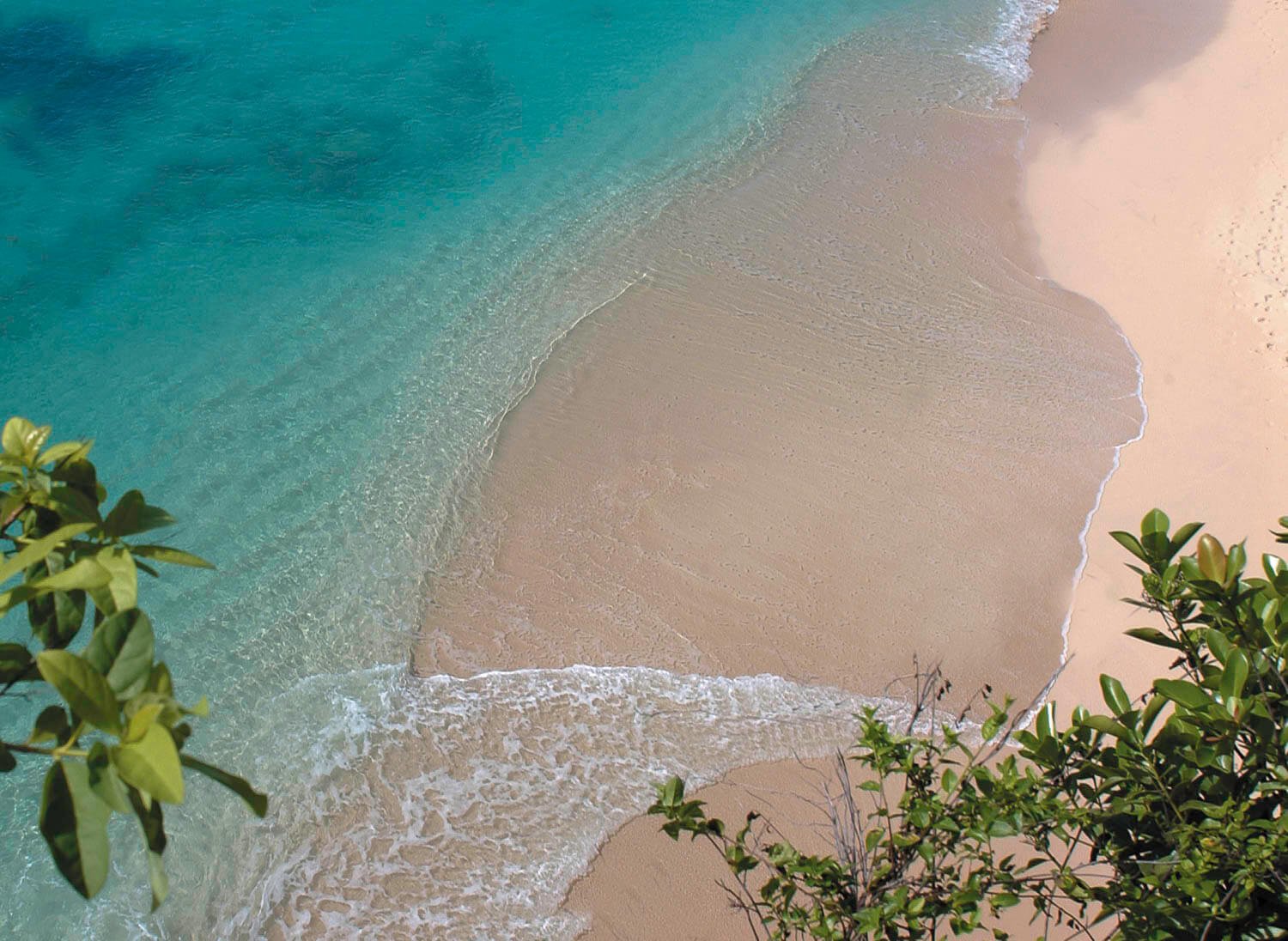This overhead aerial shot beautifully captures a tranquil beach scene. On the left side, we see clear, very pretty blue water with an almost aqua tint, progressing into areas of darker blue in the top left and center, suggesting the presence of coral beneath. As the gentle waves, topped with white foam, roll over the beach, they meet smooth, wet sand which darkens as it reaches the middle of the frame, and transitions to bright, almost peach-colored sand on the right. The soft, tan sand is peppered with footprints, hinting at recent visitors. The bottom left corner is adorned with blurred green foliage from a tree, while the bottom right showcases lush green bushes with waxy leaves, adding a vibrant contrast to the sandy shore. This serene and sunny scene, enhanced by good lighting, evokes a sense of peace and natural beauty.